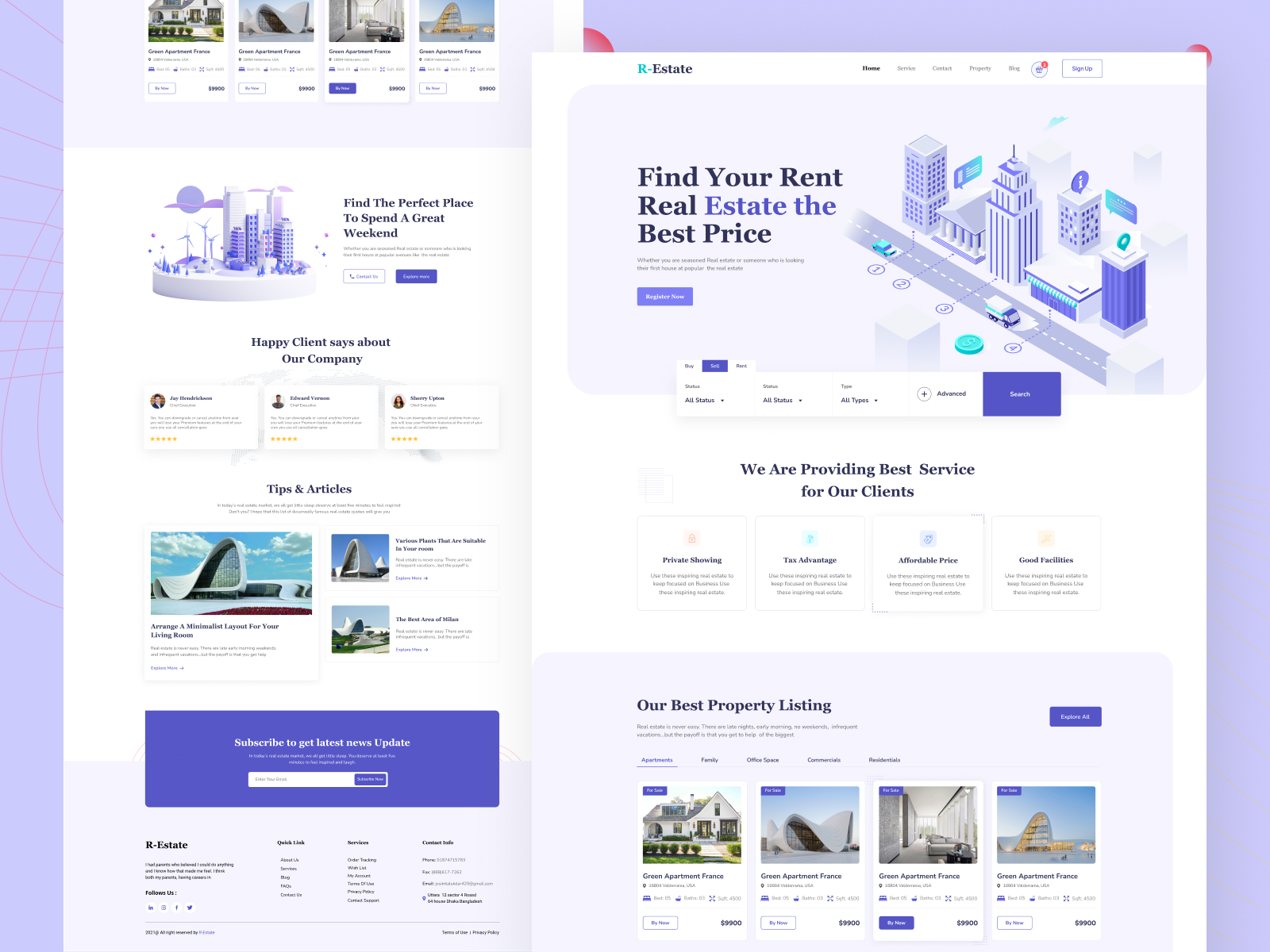On the left side of the screenshot, there's an artistic drawing rendered in shades of white, gray, and purple, depicting an intricate cityscape. To the right, the text highlights, "Find the perfect place to spend a great weekend." Unfortunately, the smaller writing below is unreadable due to blurriness. Further down, it states, "Happy clients say about our company," followed by three blurred quotes. Additional sections mention "Tips and Articles," with the writing again too blurry to decipher. The text suggests, "Arrange a minimalist layout for your living room," and discusses "Various plants that are suitable for your room" and "The best area of Milan."

On the right side, another part of an image displays headings such as "Our Estate," "Home," "Service," "Contact," "Property," "Blog," and "Sign Up." This section includes a colorful drawing in shades of blue, purple, white, and gray, showing a bustling city street lined with tall buildings and cars. The text reads, "Find to rent real estate at the best price," followed by blurred text, and "Register now." Another blurred section emphasizes their service quality: "We are providing the best service for our clients," highlighting features like "Private showing," "Tax advantage," "Affordable price," "Good facilities," "Our best property listing," and prompts readers to "Explore all." The listings predominantly feature "Green Apartment, France," repeated multiple times.